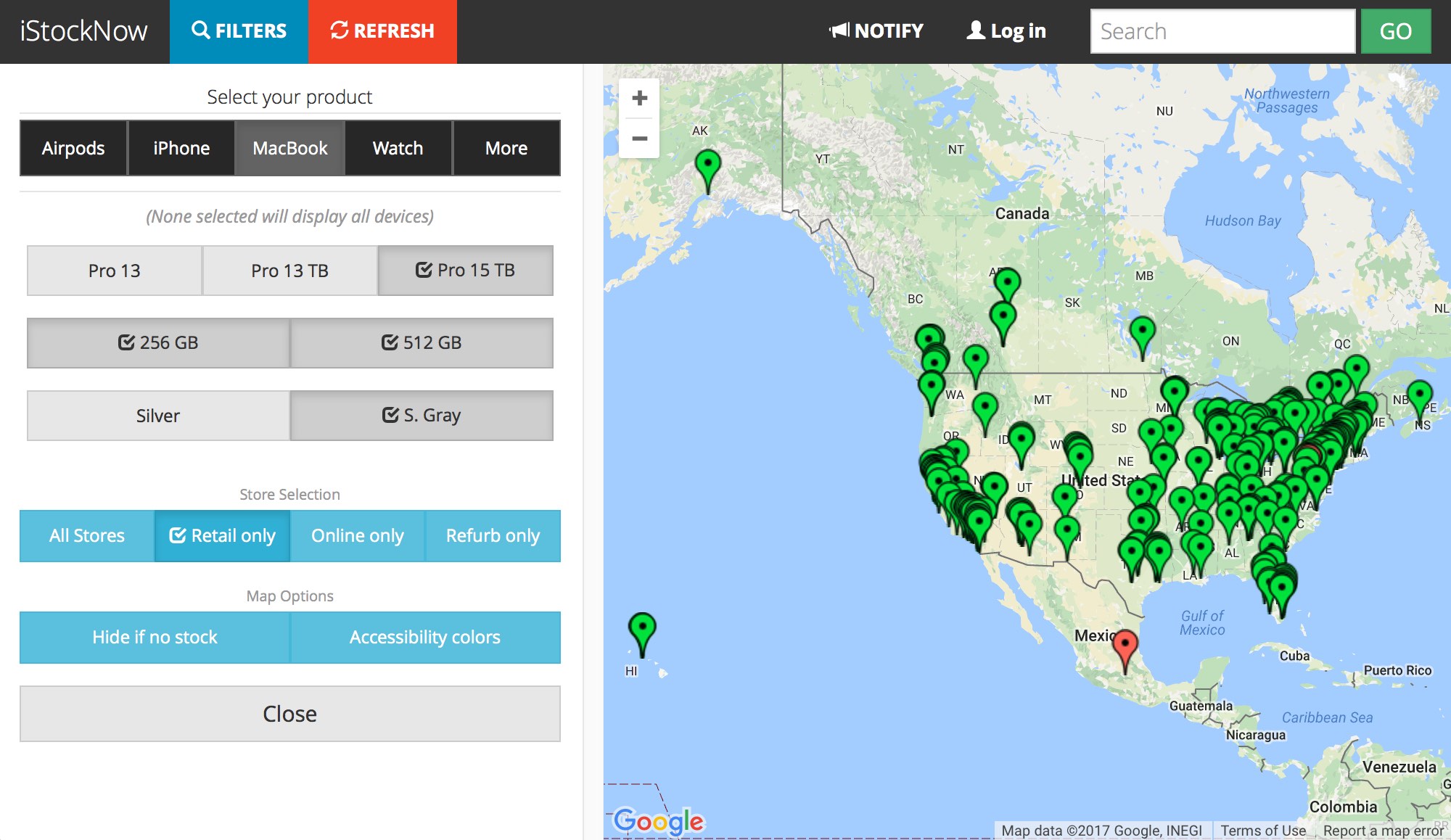A detailed caption for the described image could be:

"The image shows a webpage dedicated to listing the availability of Apple products. In the top-left corner, the page is branded with 'iStock Now'. The user interface includes options for filters, refreshing the page, notifications, and search functionalities. The user has selected 'MacBook' as their product of interest, while adjacent options for querying AirPods or iPhones are also available. A notification within the interface indicates that selecting 'None' would display all devices. Below this, several product references are displayed in individual slots. Under the 'Store Selection' options, the user has chosen 'Retail Only'. To the right of the main interface, a map of the United States is prominently featured, dotted with numerous small green flags indicating availability. Interestingly, there is a conspicuous red flag denoting unavailability in Mexico, and even an isolated green flag on a remote island presumably in the Pacific. The detailed geographical distribution suggests widespread availability across the U.S. with a few exceptions."